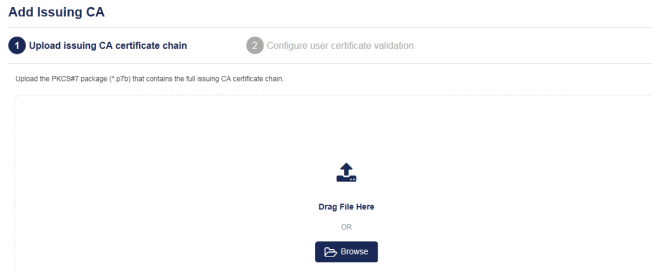The image depicts a screenshot of a user interface for adding an Issuing CA (Certificate Authority) certificate chain. 

In the upper left corner, dark blue text reads "ADD ISSUING CA." Directly below, there is a small, outlined strip with a light gray horizontal outline on the top and bottom. Inside this strip, a navy blue circle with the number "1" indicates the first step, labeled "Upload Issuing CA Certificate Chain."

To the right, another outlined area with a gray background contains the number "2" in white, labeled "Configure User Certificate Validation." Below this, small black text instructs users: "Upload the PKCS #7 package (*.P7B) that contains the full issuing CA certificate chain."

In the center of the screen, an upload icon in navy blue, resembling a disk drive with an arrow pointing upwards, is accompanied by the text "Drag file here" in blue. Below this, gray capital letters spell out "OR," and further down, a blue button with a folder icon and the word "Browse" in white offers an alternative file-uploading method.

The entire user interface is set against a plain white background.